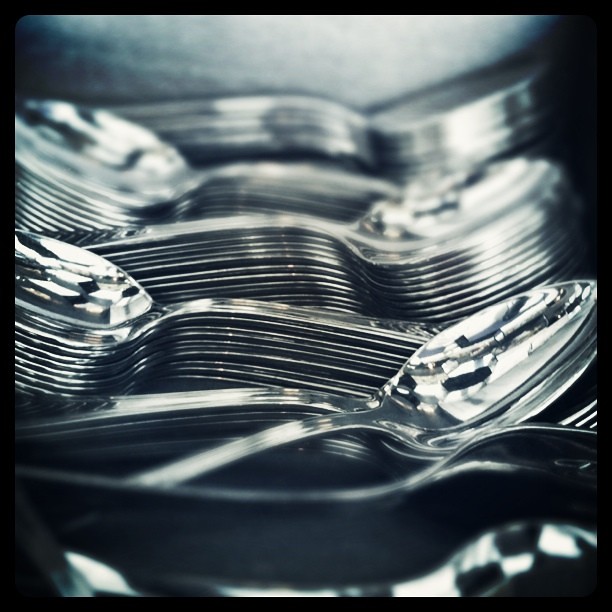In this detailed black-and-white photograph, there are six stacks of silver teaspoons neatly arranged inside a dark gray plastic container with dividers. Each stack comprises approximately eight to twenty spoons. The arrangement features an alternating pattern where the heads and bodies of the spoons shift from left to right down each stack, creating a visually intricate display with reflections that appear abstract and illusionary. The highly reflective surfaces of the silver spoons catch the light, adding to the complexity of the image. In the background, a semi-circle of light, possibly from a lamp or sunlight, illuminates the scene, highlighting the glossy texture and polished finish of the silverware. The bottom right corner of the photo reveals the lip of the container, adding depth to the composition.